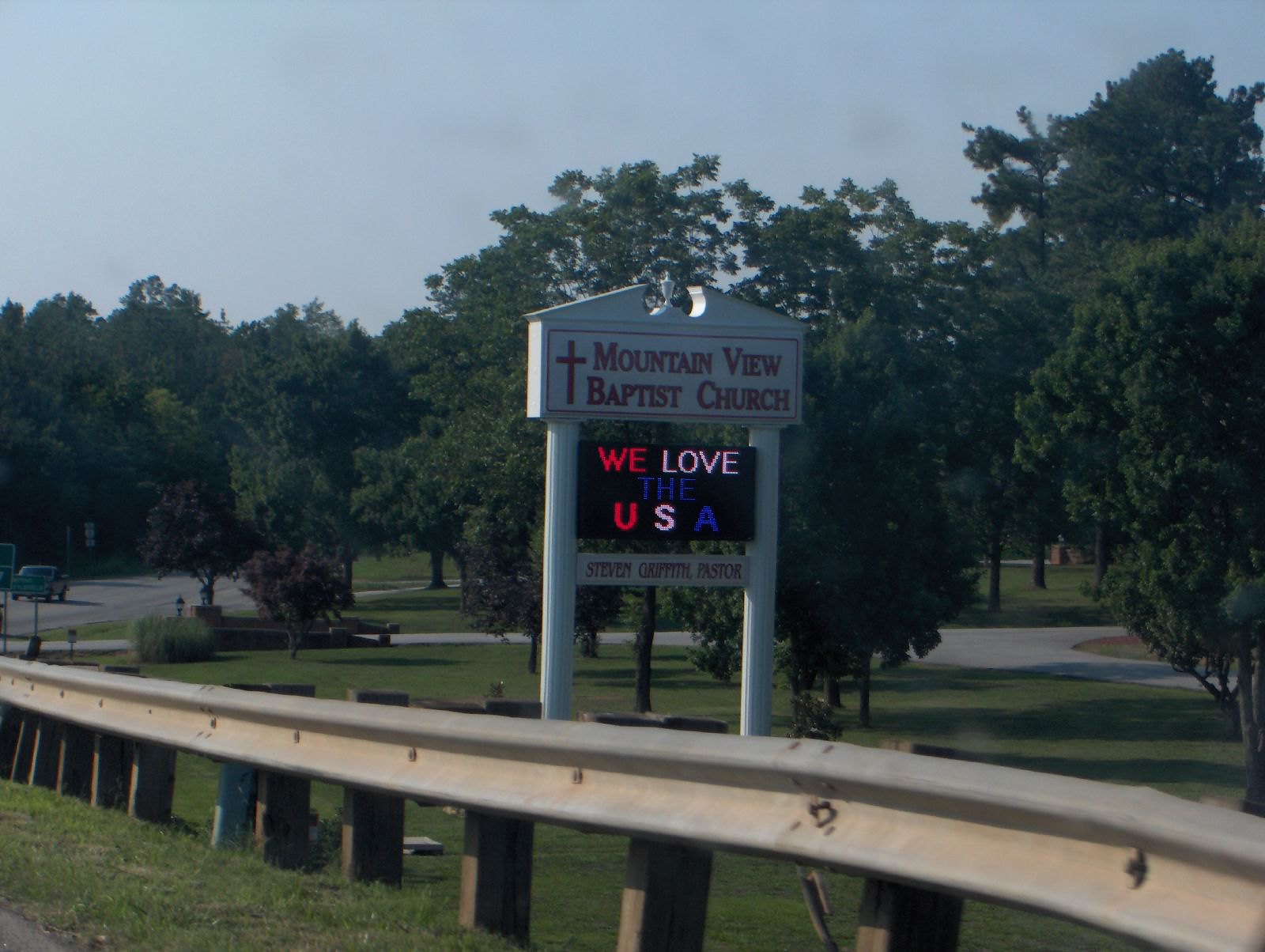Beneath a radiant blue sky on a sunny day, the grounds of a church are beautifully maintained, resembling a serene park with lush green trees and a well-kept pathway inviting leisurely strolls. The focal point of the scene is an encouraging sign, prominently displayed at the entrance, set against a foreground featuring a silver guardrail. 

The sign, with an acorn pediment at its top, introduces the location as Mountain View Baptist Church. It features an eye-catching design, with "Mountain View Baptist Church" written in dark red lettering, accompanied by a cross on the left-hand side. Below this, a digital section stands out with a patriotic message: "We Love the USA," where "We" is in red, "Love" is in white, "The" in blue, and "USA" in a mix of red, white, and blue.

Additional detail on the sign includes the name of the pastor, which is partially obscured but begins with "Stephen." The sign is supported by white posts, completing the inviting and encouraging atmosphere of the church's welcoming grounds.